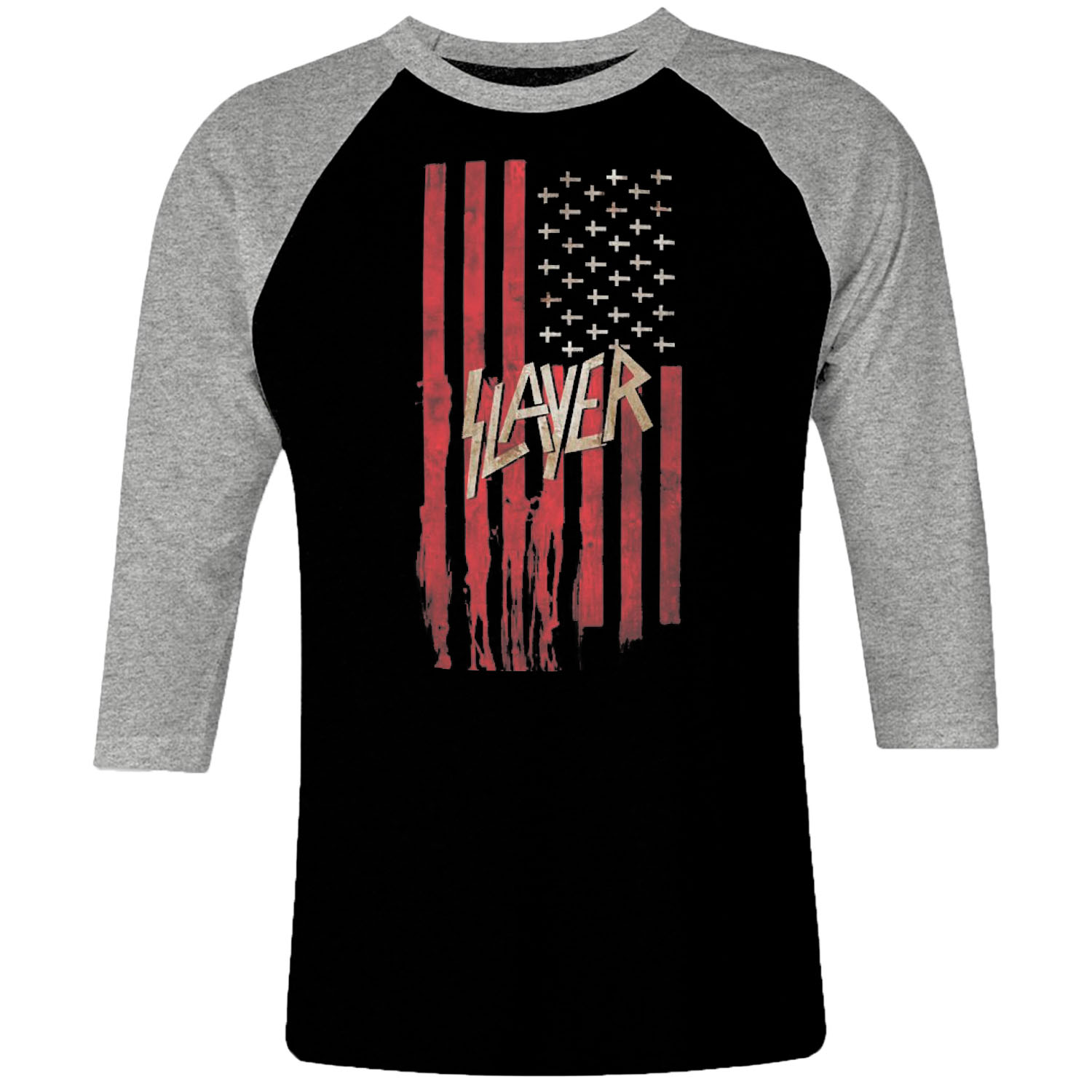This image features a three-quarter length Henley-style t-shirt displayed on a white background, typical for retail sites. The shirt has gray sleeves extending to just below the elbows, and a matching gray ribbed neckline. The body of the shirt is black. Prominently displayed on the front center is a vertical American flag, but with distinctive elements: the stars are replaced by inverted crosses, and the traditional blue field is rendered in black. The flag's stripes are a mix of red and black, extending downward in a frayed, worn design. Superimposed on the flag is the word "SLAYER," written in a jagged, lightning bolt-like font that's evocative of heavy metal aesthetics. The flag and lettering give a bold, distressed look to the shirt, with no indication of its intended gender audience.